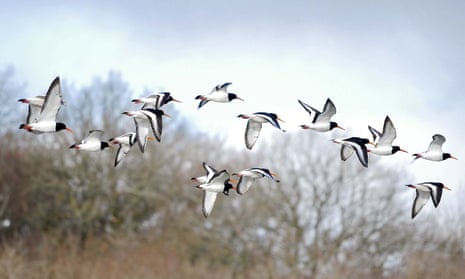In this color photograph taken during the daytime, a flock of approximately 14 birds can be seen flying from left to right. The birds, which are medium-sized with black heads, necks, and wingtips, also feature white chests and bellies. The upper portions of their wings are black with a distinct white band along the edge. The scene is captured from ground level looking up, allowing for a full view of the birds' flight against a sky that transitions from blue and white near the horizon to gray higher up. Below the birds, the landscape is filled with trees that vary in appearance; on the left, the trees still have spots of green and brown leaves with a dusting of snow, while on the right, the trees are mostly bare. The overall composition of the image presents a realistic representation of nature, blending the dynamic movement of the flock with the stillness of the wintry trees.